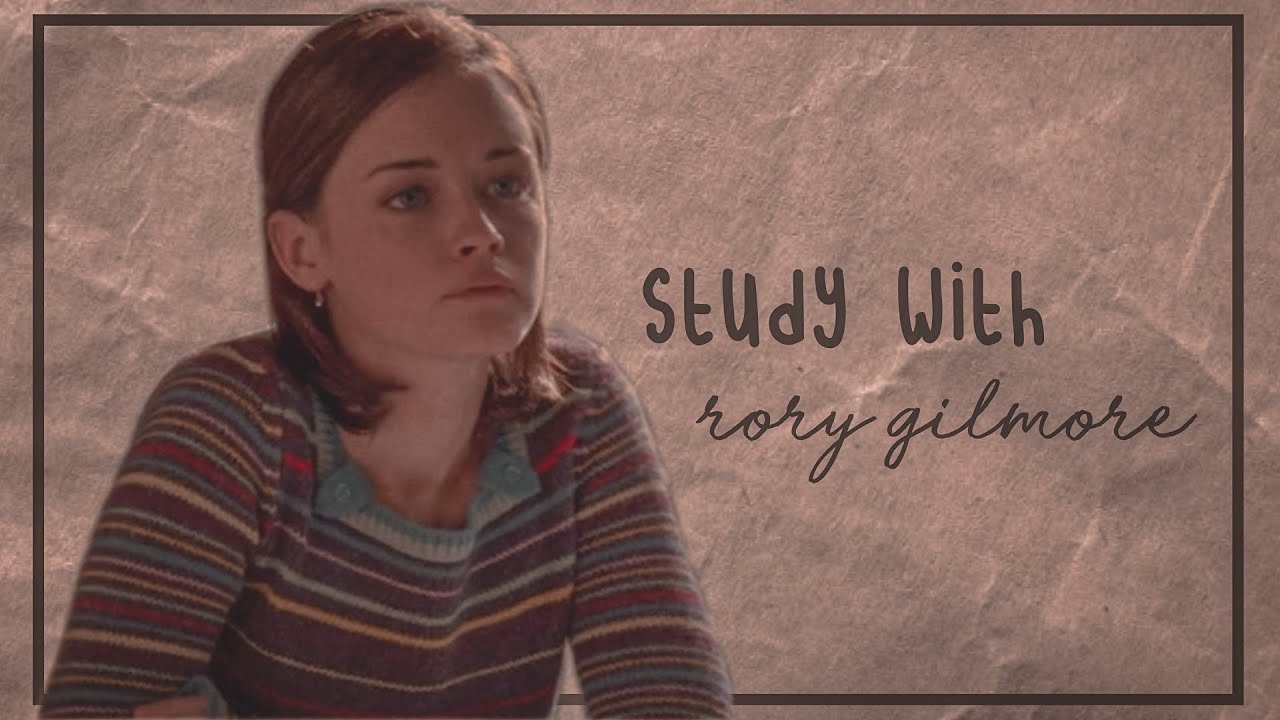The advertisement for the TV show "The Gilmore Girls" features a rectangular image with a crumpled brown paper backdrop, bordered in black. On the left side, there's a picture of Alexis Bledel, the actress who plays Rory Gilmore. She has short, shoulder-length brown hair tucked behind her ears and striking blue eyes. She is depicted leaning slightly forward in a three-quarter profile with a neutral expression. She wears a predominantly maroon sweater with thin stripes of white, red, yellow, and light blue. To the right of her image, the text "Study With Rory Gilmore" is displayed, with "Study With" in a playful print font and "Rory Gilmore" in elegant script.